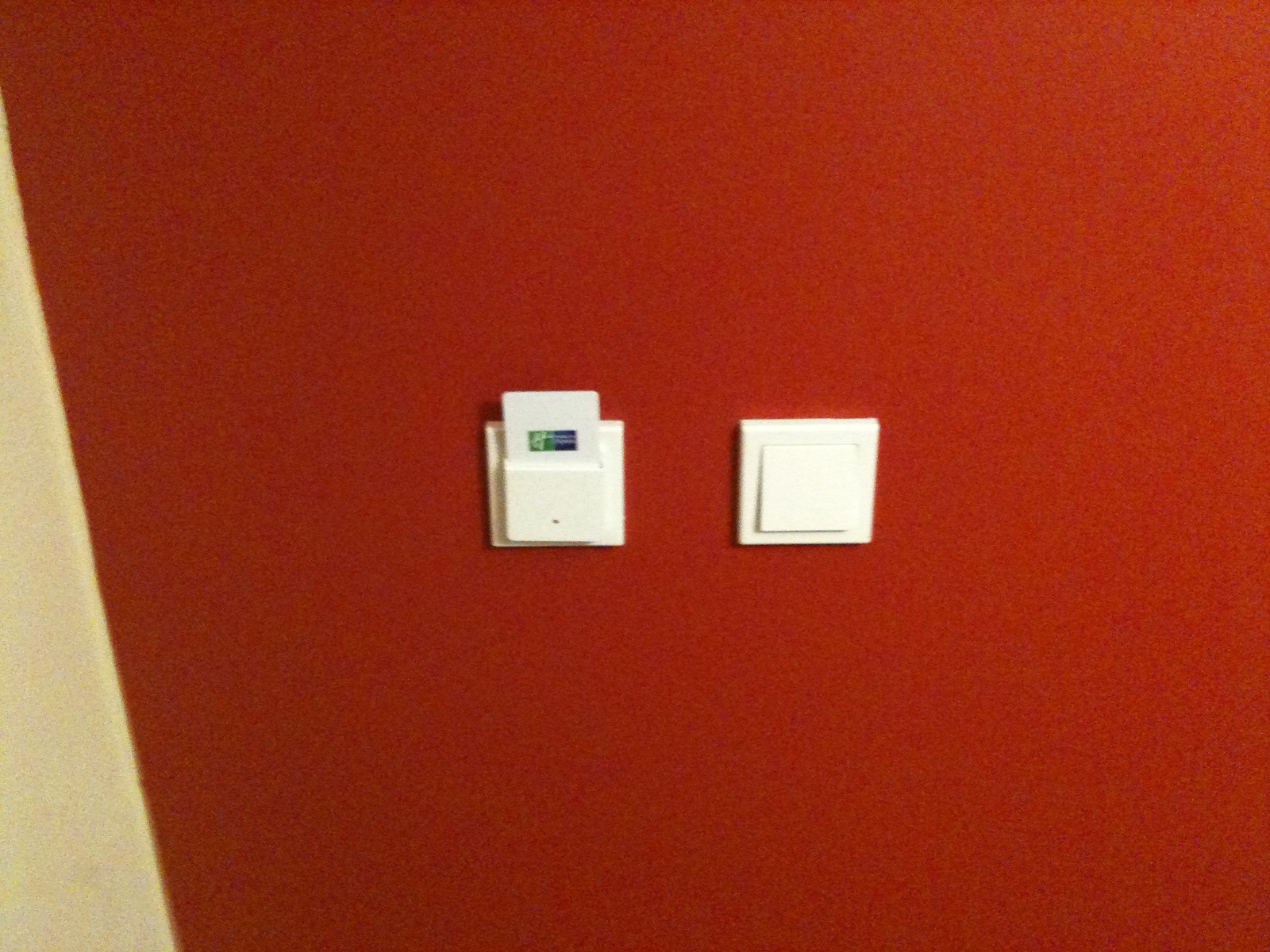The image depicts a dark brick or terracotta-colored wall abutting a paler beige wall. Centrally positioned on the wall are two white square patches, presumably switches. Unlike typical UK rocker switches, these switches exhibit minimal raised surfaces, resulting in an overall flat appearance. However, slight shadows indicate a subtle elevation, particularly on the right-hand switch. The left-hand switch features a raised area at the top, adorned with an image and text that are too small to be discernible. These switches likely serve an interior function, although their exact nature remains unclear.